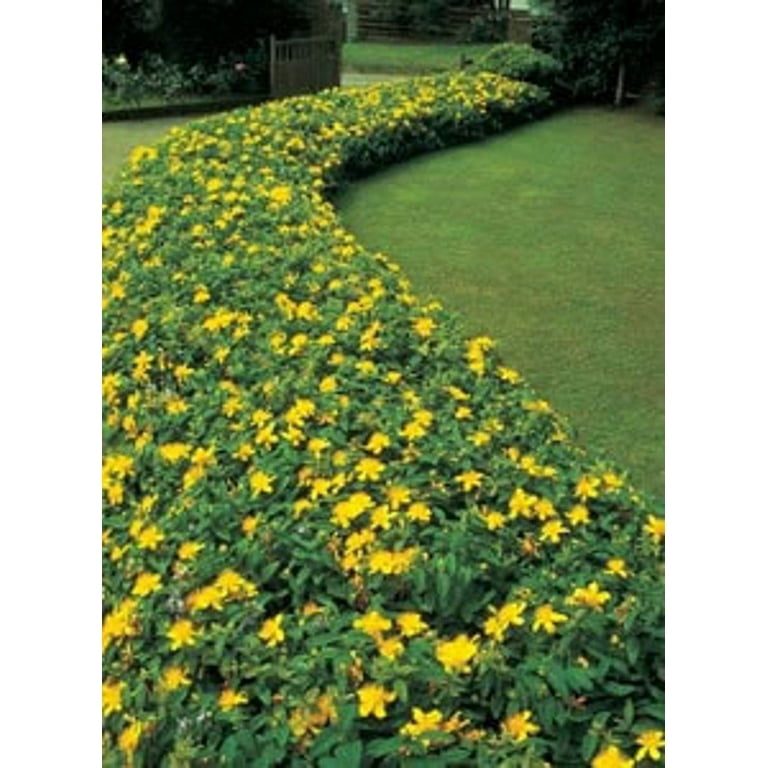The image captures a meticulously manicured garden scene, dominated by a vibrant hedgerow teeming with small yellow flowers, each boasting four to five delicate petals. This hedge forms a semi-circle, curving slightly to the left and forward, before veering to the right. Flanking the hedge on both sides is a well-maintained, lush green lawn, trimmed to perfection. In the upper part of the image, an open metal gate stands slightly ajar, leading to a different section of the yard. The background hints at more well-tended greenery and possibly a building, adding depth to the serene garden setting. Bright yellow and green hues predominantly color the scene, highlighting the orderly beauty of this tranquil space.